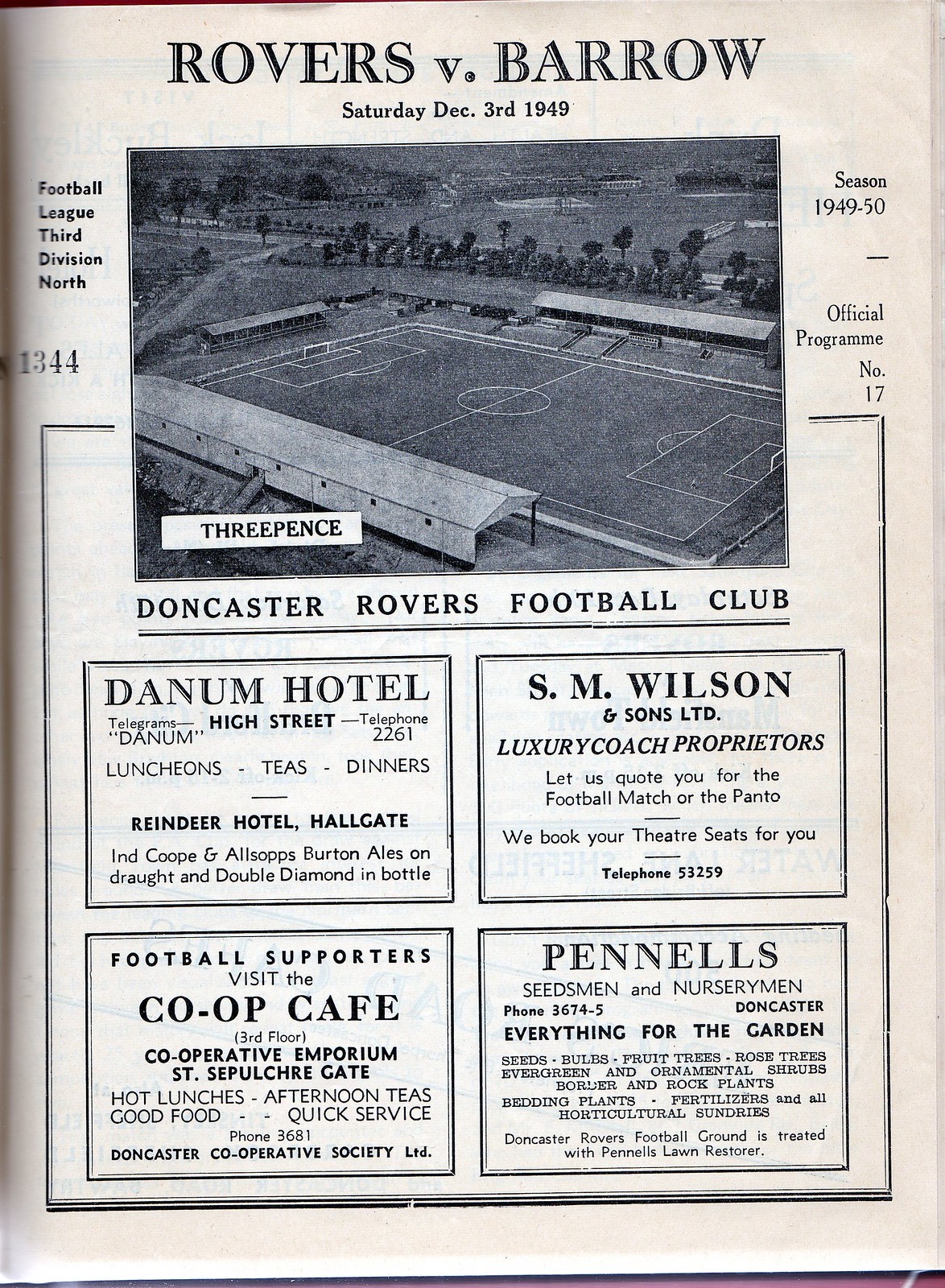This vertically aligned rectangular image depicts a page from a 1949 newspaper or sports journal, featuring a black and white photograph of a soccer field with trees in the background and no players visible. The headline, "Rovers versus Barrow," is written in all caps, black letters, followed by the date, "Saturday, December 3rd, 1949," in smaller black print. To the left of the photo, there's a label indicating "Football League 3rd Division North," while to the right, the page mentions "Season 1949-50, Official Program No. 17." Below the photograph, the text reads "Doncaster Rovers Football Club," suggesting the location is Doncaster, possibly in the UK. The bottom section of the page contains four square advertisements for local businesses: the "Danum Hotel," "S.M. Wilson and Sons Limited," "Football Supporters Visit the Co-op Cafe," and "Pennell's Seedsmen and Nurserymen," arranged in a grid format. The overall composition and details imply this is an official program page reporting on a football (soccer) match and related local advertisements.